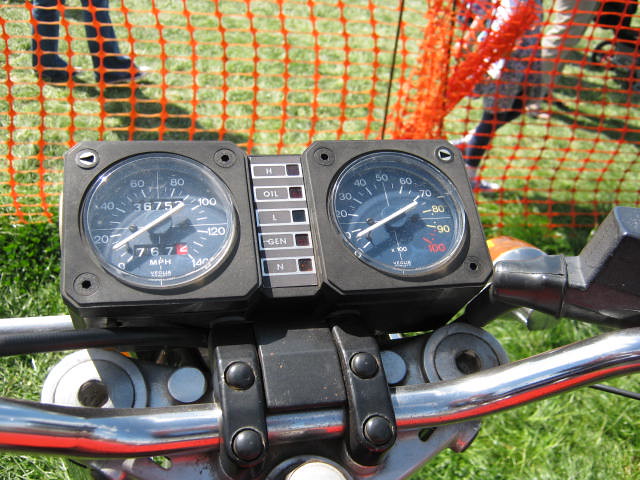The image captures the handlebars and instrument panel of a powered two-wheeled vehicle, possibly a moped or dirt bike, against a backdrop of a grassy area. The focus is on the black, square-shaped housing containing two circular gauges side-by-side; one appears to be a speedometer in miles per hour, while the other seems to be an RPM gauge, both with numbered indicators and hands. Beneath the gauges, there are five vertically aligned indicator lights, each labeled with different letters: 'H', 'oil', 'L', 'gin', and 'N'. Surrounding the vehicle, on the ground, is a stretch of green grass and an orange plastic netting, resembling a temporary fence. Behind this fence, only the legs of several people are visible, suggesting they are standing or moving around nearby.